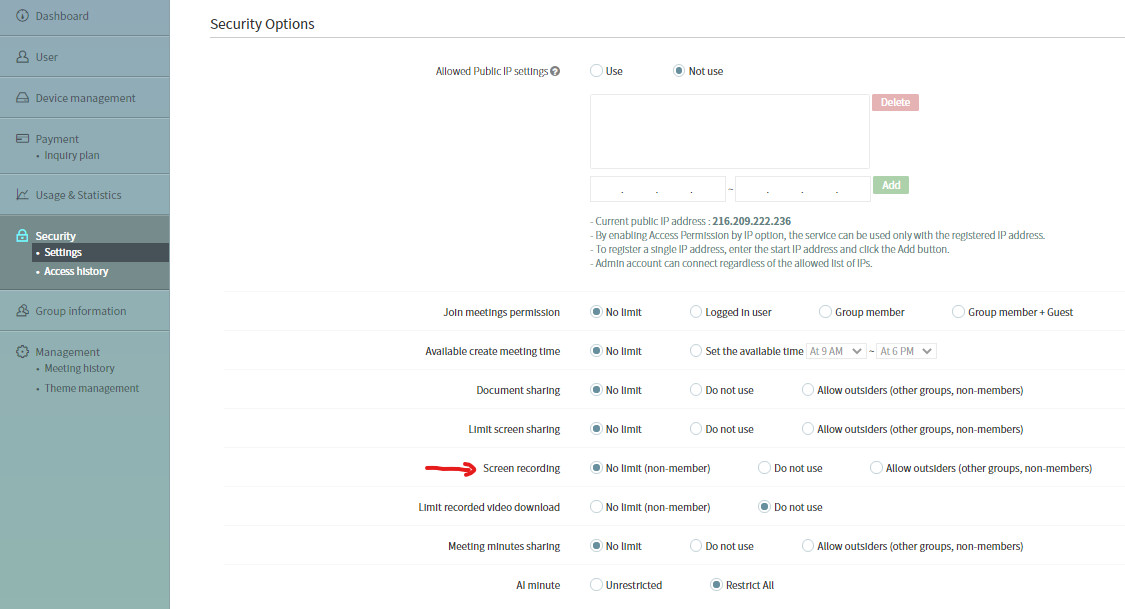The image is a color screenshot taken from a software interface, most likely an administrative dashboard. On the far left, there is a vertical navigation panel containing various menu options. At the top of this column is the "Dashboard" option, followed by "User," "Device," "Payment," "Inquiry," "Plan," "Usage and Statistic," and "Security." Under the "Security" section, additional sub-options are listed which include "Settings," "Access History," "Group Information," "Management," "Management History," and "Fee Management."

To the right of this navigation panel, the main area displays the security settings. At the top, there is a toggling option labeled "Allowed Public" with two choices: "Use" and "Not Use," the latter of which is currently highlighted. Below this, there is an empty text box labeled "Current Parameters," followed by a list of security permission settings, each accompanied by their respective current states. These settings include:

- Permissions: No
- Available Time: No
- Document Sharing: No
- Limit Screen Sharing: No (highlighted with a red arrow pointing to it)
- Screen Monitoring: No
- Limit Download: Do Not Use
- Marketing Sharing: No
- All Minute: Restrict All

The screenshot provides a comprehensive view of the software's security configuration, with emphasis on the specific restrictions and permissions in place.